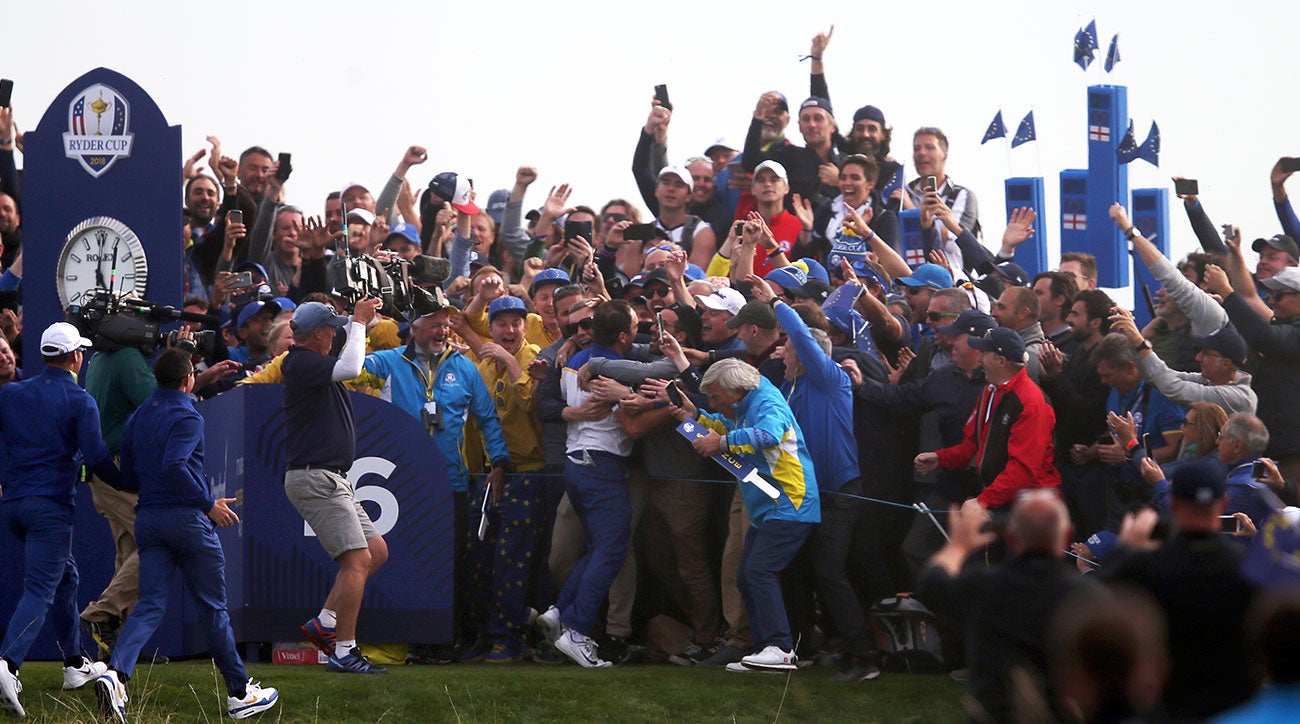This is a jubilant outdoor photograph celebrating the Ryder Cup at a golf venue. A large group of enthusiastic people stands at the center, many with their hands raised, smiling broadly. Several men in the front are seen embracing each other in heartfelt hugs, while others are waving small flags. Their attire varies, with most wearing jackets, and a few capturing the moment with their phones. To the left, more people are walking towards the central group. Prominently to the left side of the image, a tall board rises above the crowd, displaying the Ryder Cup emblem in blue, white, and gold. Just below the emblem is a large clock with a silver frame and Roman numerals, adding a classic touch to the scene. The backdrop features a light blue sky with scattered clouds, hinting at a pleasant day for the event.